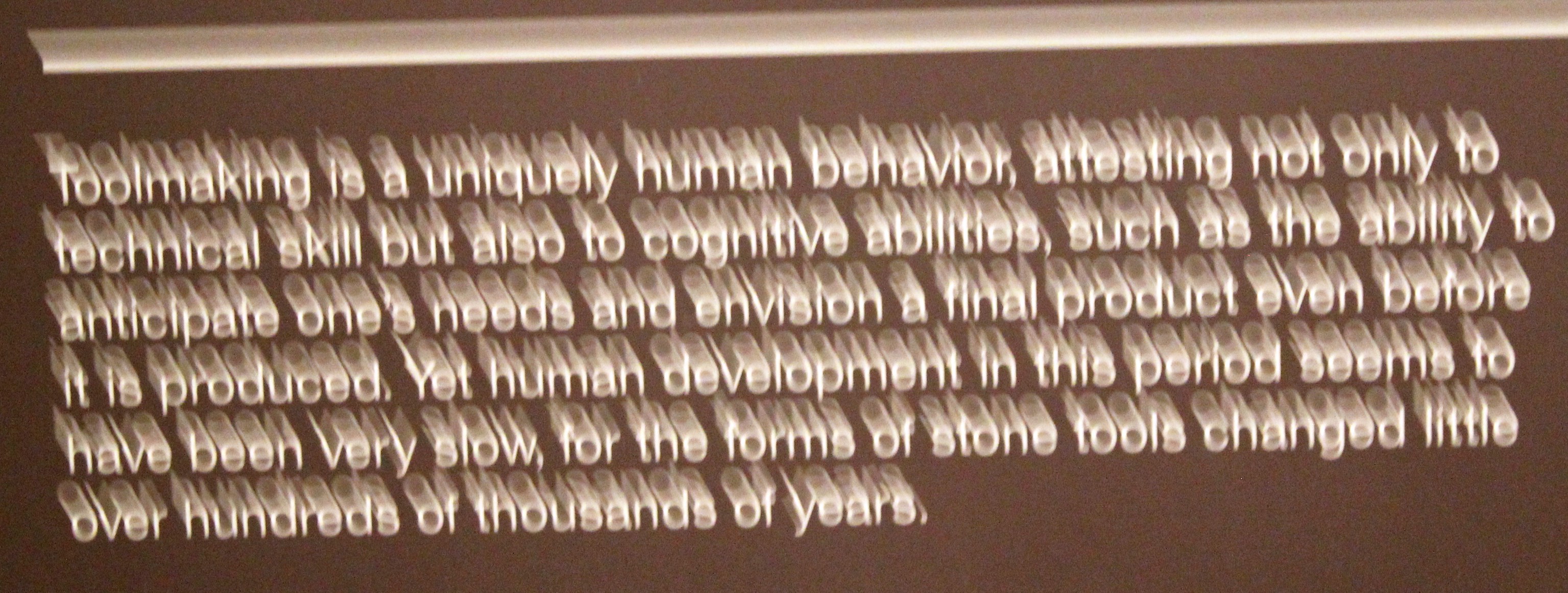The image portrays a photograph or scan of a paragraph of text set against a dark brown background. The text, in a white or creamy font, displays a severe ghosting effect, creating a translucent, stretched duplicate of each letter, giving a three-dimensional and blurred appearance. The text reads: “Toolmaking is a uniquely human behavior, attesting not only to technical skill, but also to cognitive abilities, such as the ability to anticipate one's needs and envision a final product even before it is produced. Yet human development in this period seems to have been very slow, for the forms of stone tools changed little over hundreds of thousands of years.” There is a light gray, horizontal piece of conduit or plastic running along the top of the image, unaffected by the ghosting effect, suggesting the blurring might be a digital effect applied exclusively to the text.